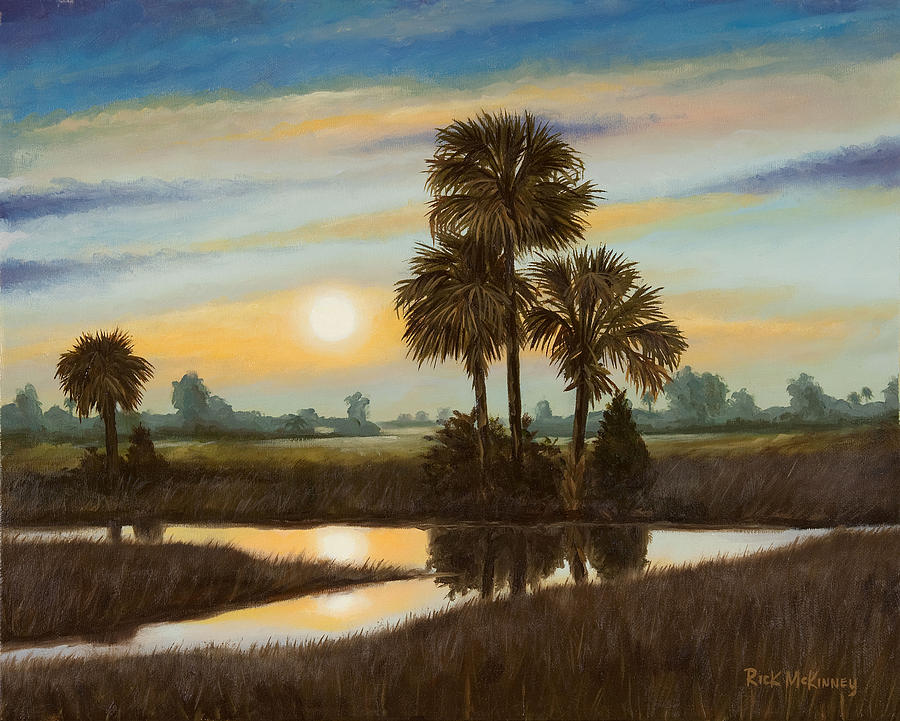This vibrant painting, created by artist Rick McKinney as indicated by his handwritten signature in the lower right corner, captures a serene tropical marshland at either sunset or sunrise. The sky is an array of striking colors, transitioning from dark blue at the top to light blue, orange, and finally yellow near the horizon, where a pale white sun hovers, casting a gentle halo and reflecting in the water below. 

Dominating the middle ground are four prominent palm trees—three positioned centrally and one slightly to the left. The landscape, brimming with lush grass, reeds, and smaller trees and bushes, frames a meandering waterway that forms a backward L-shape and ends in a V towards the left. The perspective reveals a layered composition, with distant trees silhouetted against the horizon, providing a sense of depth and tranquility. The scene's detailed portrayal of water, vegetation, and sky captures the essence of a vibrant, peaceful evening or early morning in a tropical setting.